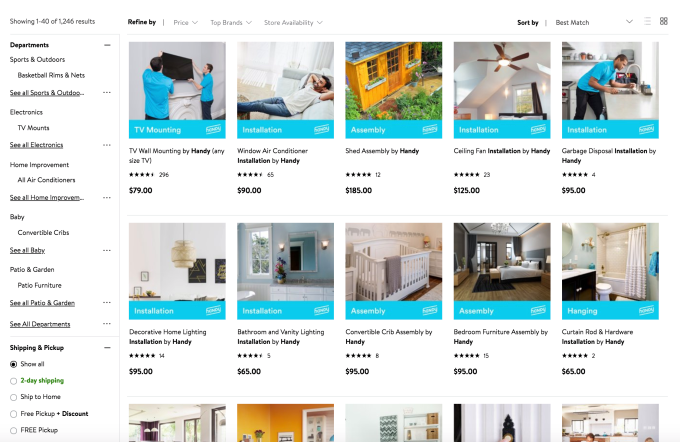The image, albeit slightly blurry, depicts an online marketplace interface where users can purchase or install various home improvement services or items. At the top of the screen, it prominently displays "Shopping: 1 out of 40 results" alongside a "Refine by" option for filtering the results. The central portion of the screen features a grid of photos arranged in a layout with five images horizontally and approximately two and a half images vertically. 

Each photo showcases either a home installation in progress or the finished product, accompanied by a blue banner at the bottom. The first banner reads "TV Wall Mounting" and denotes "Buy Handy Gary" in black font, giving a possible indication of the service provider. Below each photo, although somewhat blurry, there appears to be pricing information. 

Notable images include:
1. Two men in blue shirts mounting a TV.
2. A person lounging on a couch.
3. A ceiling fan.
4. A man in a blue shirt working on a sink.
5. Various other domestic settings.

These photographs collectively illustrate diverse services available for home improvement, each marked by distinct visuals and pricing details.